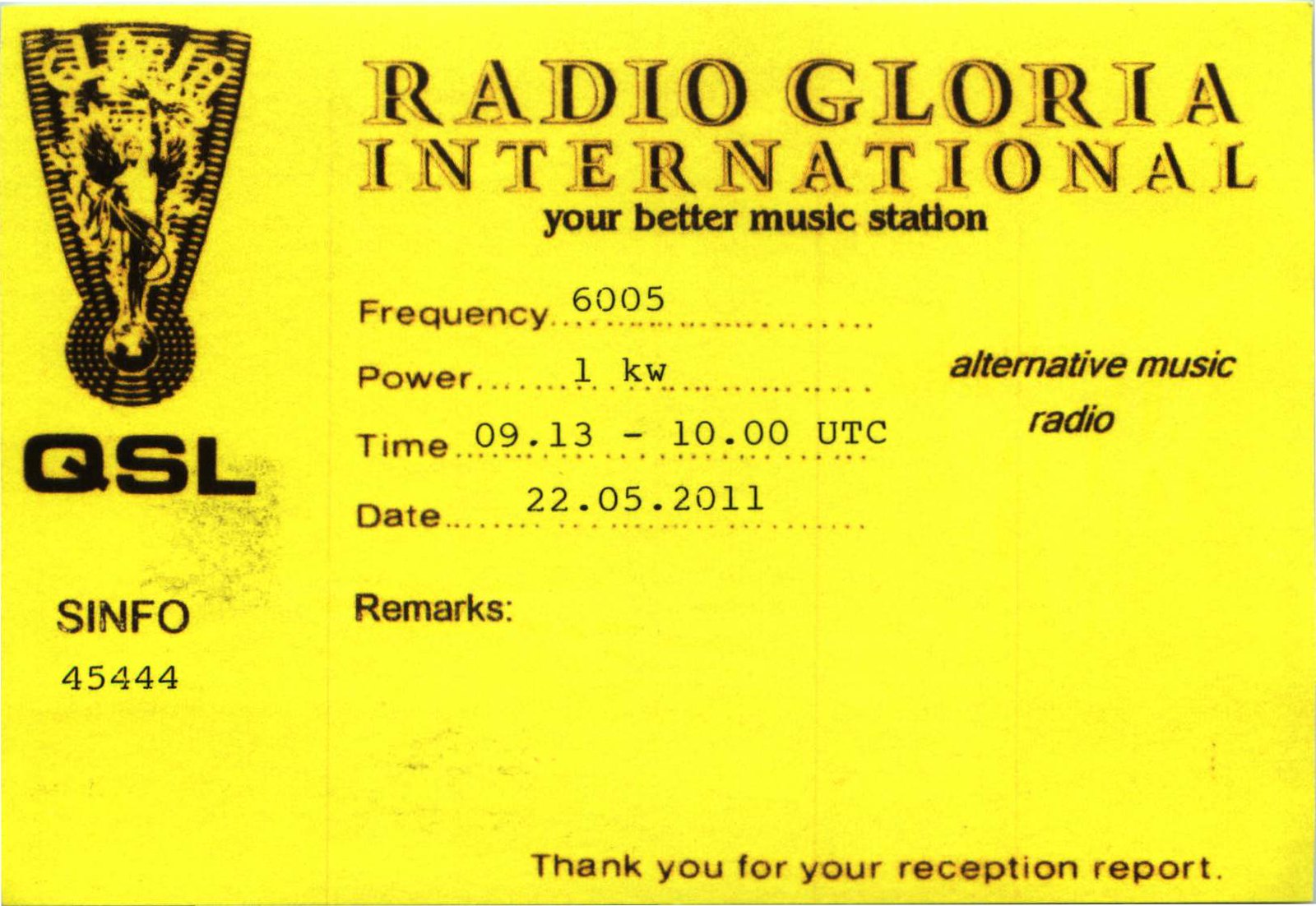The image depicts a horizontal rectangular advertisement for Radio Gloria International. The background is a bright yellow with brown lettering prominently displaying the station's name at the top: "Radio Gloria International". Below it, in black letters, is the tagline "Your Better Music Station". The advertisement includes detailed information: Frequency is 6005, Power is 1 kilowatt, Time is 09.09.13-10.00 UTC, and the Date is 22.05.2011. To the right, in brown letters, it states "Alternative Music Radio". A notable symbol appears off to the left, resembling an upside-down triangle with a rounded bottom, beneath which "QSL" in large black letters is visible. The text is followed by "Remarks: thank you for your reception report" and "SINFO 45444". The advertisement appears somewhat dirty, suggesting it might be a rough copy or old print.